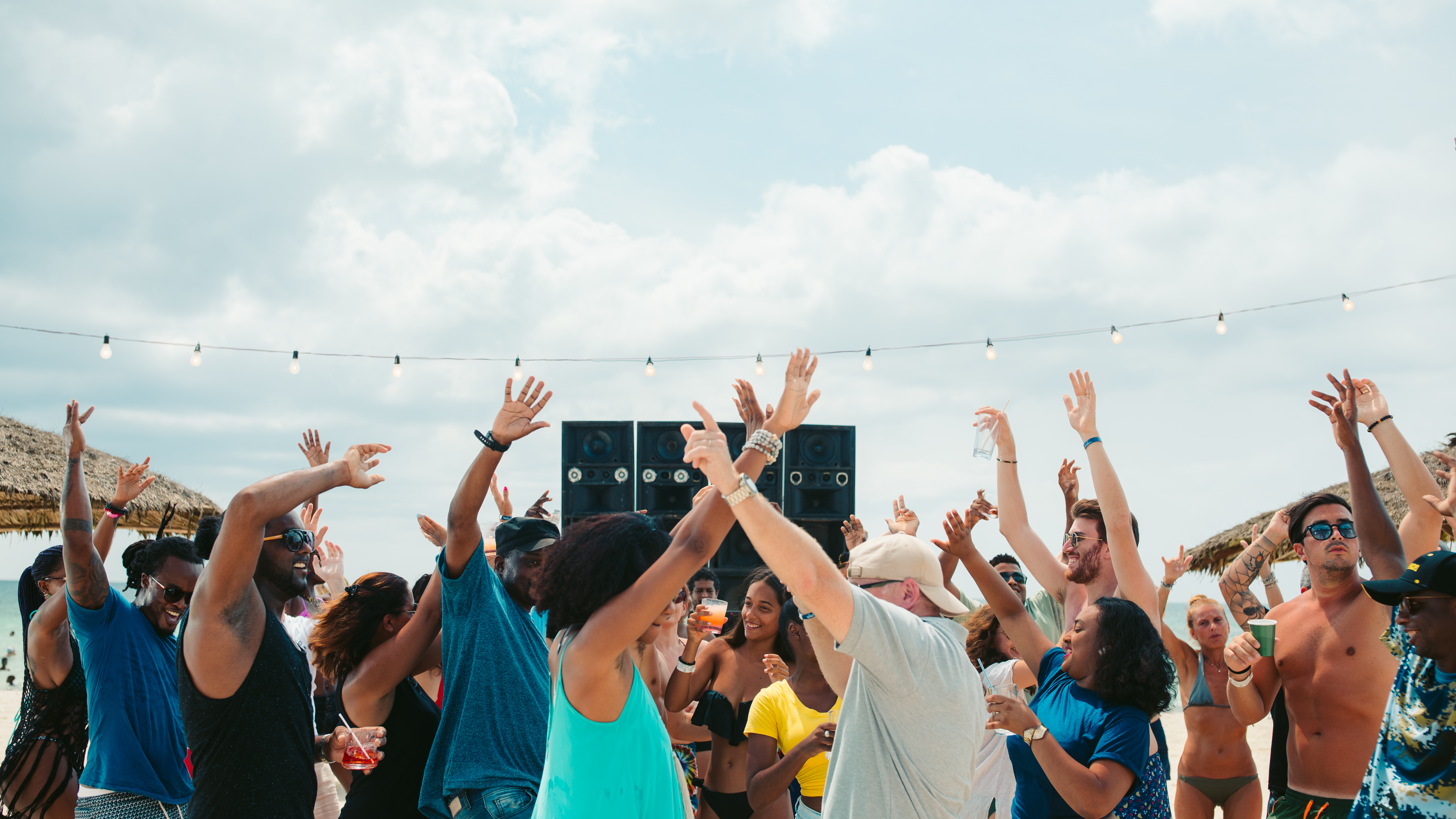This vibrant photograph captures a lively beach concert or party scene during the day, set against a serene backdrop of a light blue sky dotted with fluffy white clouds. The foreground is dominated by a diverse crowd of people, roughly 20 in number, who are fully immersed in the festivities, many with drinks in hand. Most revelers are dressed for the warm weather, in swimsuits, bikinis, or light summer clothing, with numerous individuals bare-chested. Almost everyone's arms are raised in the air, creating an energetic and unified display of joyous celebration. 

In the center of the image, a striking focal point shows a black woman in a teal sleeveless shirt beside a white man in a gray shirt and a white hat, their arms intersecting as they dance. Above the throng, a string of evenly spaced white lights stretches across the scene, adding a festive ambiance. Peripherally, thatched roof beach huts and a set of large black speakers can be seen, enhancing the celebratory beach environment. The scene exudes a sense of unity and shared happiness, with smiles and music contributing to the electrifying atmosphere.